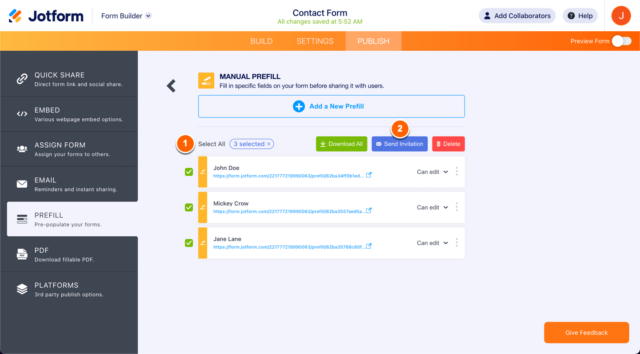The image features a user interface with a gray background displaying the JotForm Form Builder. Prominent elements include a gray oval with the label "Add Collaborators," accompanied by another gray oval labeled "Help," distinguished by having a question mark. Additionally, there is an orange circle containing the letter "J" in white.

On the left side, a gray vertical rectangle is visible, listing various options such as Quick Share, Embed, Assign Form, Email (highlighted in white), Prefill, PDF, Platforms, and Manual. A blue rectangle appears within this sidebar, featuring a white plus sign inside a circle and labeled "Add a New Prefill." 

A functional description next to this element reads "Fill in specific fields on your form before sharing it with users." Moreover, a selection option displays a numeral "1" beside "Select All," indicating one item has been chosen. Nearby is an oval marked "3 selected," and a green rectangle containing a down arrow with the instruction "Download All."